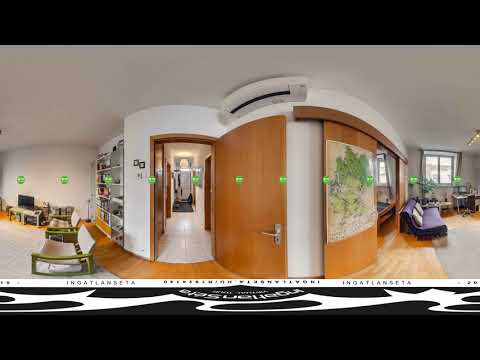The image showcases a distorted, panoramic view of an indoor setting that appears to be a mix between an office and a living room, with the image bowing towards the viewer in a U-shape. The room has white walls and a light wooden floor. On the left, there's a collection of furniture creating a sitting area. This area includes green and tan pieces, possibly chairs and a sofa, with a black TV screen positioned on the far left corner. Further towards the left center, there's an open doorway leading to another room.

On the right side, there is a seating area featuring a purple, low couch alongside other pieces of furniture. This side also has shelves filled with various unidentified objects. There's a window positioned near this area, allowing a view outside. A section of the wall on the right displays an image that looks like a map with green and brown sections. The floor in this corner is partially covered by a gray rug.

The central part of the image features a brown wooden door that is bent due to the distortion effect. This door acts as a focal point, emphasizing the room's stretched perspective. The entire image is framed with thick black borders at the top and bottom, adding to the visual distortion.